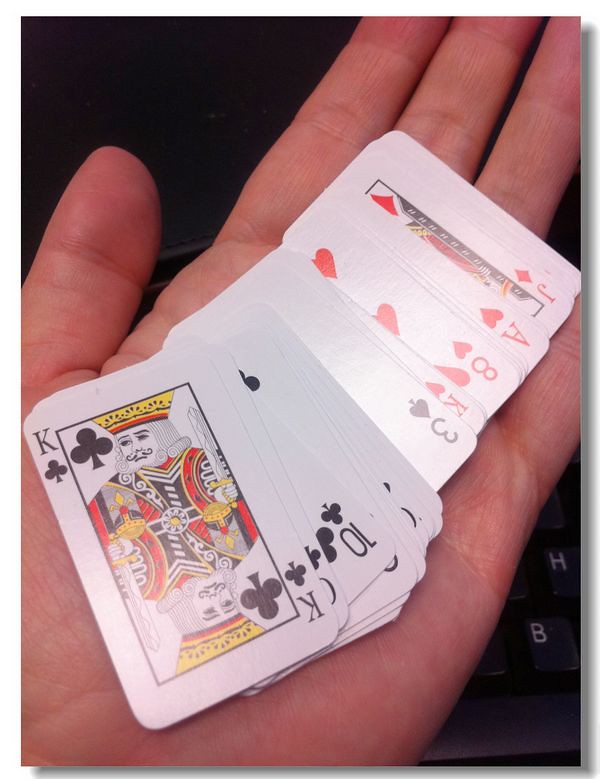In this color photograph, a left hand is seen palm-up, positioned so that the wrist is in the lower left corner while the fingertips extend to the upper right corner of the portrait-oriented frame. The tips of the fingers are cut off, but the knuckles of the fingers and most of the thumb are visible. Resting sideways in the hand is a deck of miniature playing cards, each approximately two to two and a half inches tall, fanned out and held face-up. 

A light source shines down from the top right, illuminating the cards and casting soft shadows. Below the hand, a black computer keyboard is partially visible, with the spacebar and keys like 'B' and 'H' clearly seen.

The cards displayed include the King of Clubs, a partially obscured club card, the Ten of Clubs, and several other club cards that are overlapped. In the brighter area of the photo, the Three of Spades, King of Hearts, Eight of Hearts, Ace of Hearts, and Jack of Diamonds are discernible. The remaining cards are hidden by the overlapping arrangement of the deck.